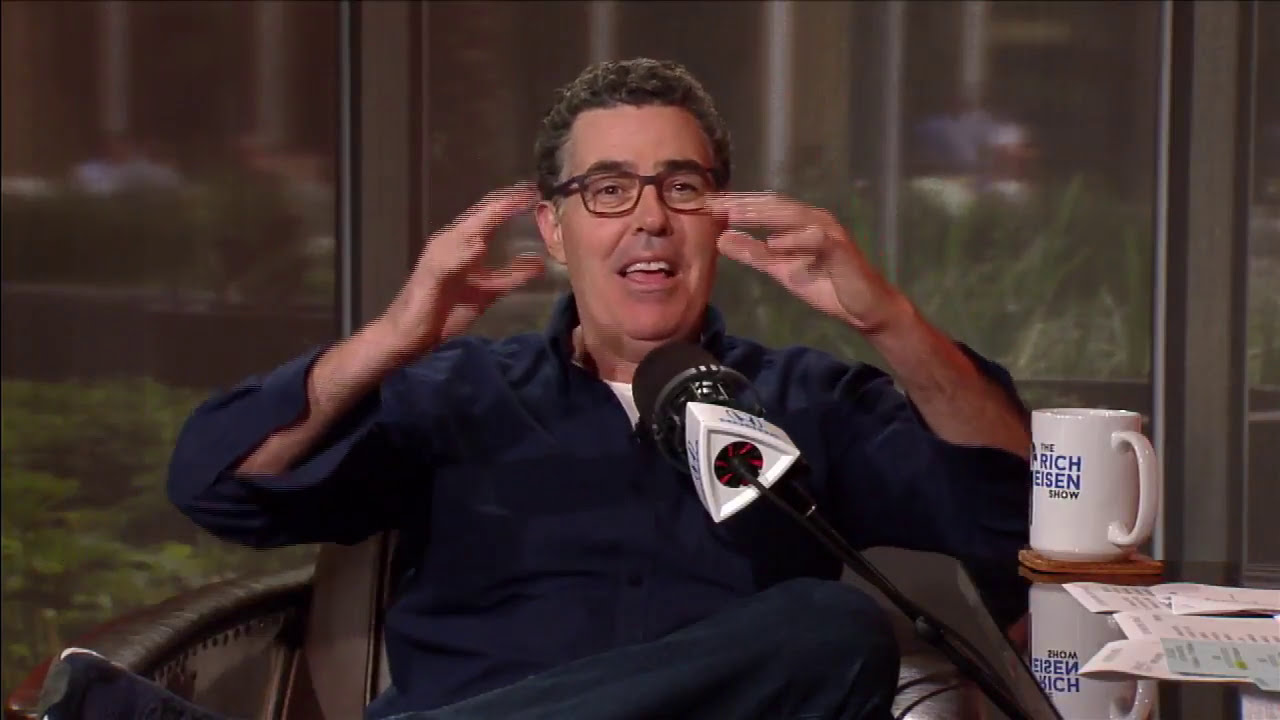This horizontal rectangular image features a man seated and engaging with a microphone. He has short, curly black hair and is wearing distinctive red glasses. His mouth is open in mid-sentence, revealing his top teeth and suggesting he is speaking while conveying a point with his blurred, raised hands. He is dressed in a navy blue, long-sleeve button-down shirt, possibly over a white t-shirt, and black pants. The background is somewhat blurry but reveals large windows with brown borders that offer a view of greenery, including grass and some plants. The man is seated in what appears to be a chair with a brown cushion. In front of him rests a white coffee mug emblazoned with "The Rich Eisen Show" in blue and black letters; next to the mug is a messy stack of papers. A notable detail is the black microphone with a white base, positioned centrally in front of him, adorned with the Honda logo, signifying he might be part of a podcast or talk show setup.